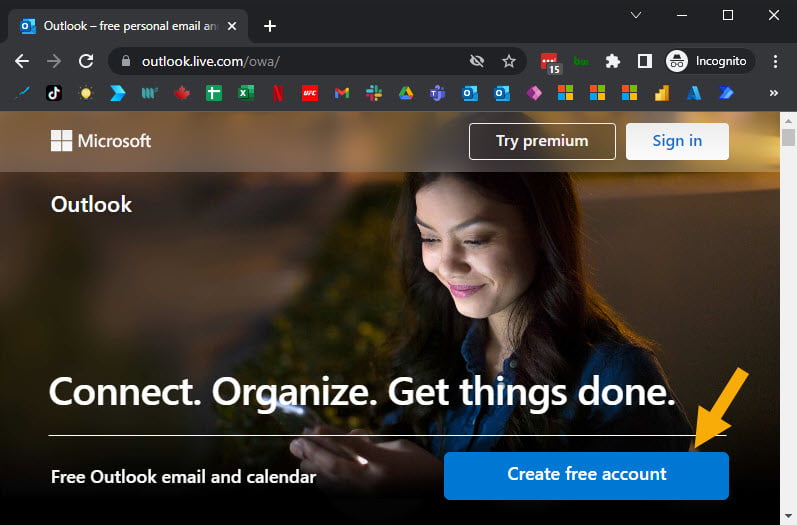Screenshot of the Microsoft Outlook Website Interface:

In the upper-left corner of the screenshot, against a gray background, the text reads "Outlook - Free Personal Email." The top border of the interface is black, featuring a white plus sign meant for adding a new tab. 

To the right of the new tab button, there are the minimize, maximize, and close window buttons. Below this, a navigation bar includes a back arrow, forward arrow, and a refresh button. The URL displayed reads "outlook.live.com/owa/" with a hidden eye symbol indicating private or incognito mode, and a favorites button adjacent to it. The far-right section of the navigation bar features an incognito mode icon and an extensions button.

Further down the interface, various icons for different applications can be seen, including those for brightness adjustment, TikTok, Netflix, UFC, Gmail, Google Drive, and several Microsoft applications.

Prominently placed is the Microsoft logo and name in white text, alongside a "Try Premium" button and a "Sign In" button. Below this header, the large text reads, "Outlook: Connect, Organize, Get Things Done." Accompanying this text is a blue button labeled "Create Free Account," highlighted by a yellow arrow pointing towards it.